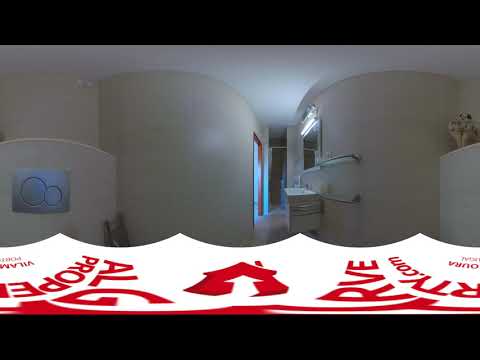This image is a panoramic indoor scene likely taken with a 360-degree camera lens, creating a slightly distorted effect where the walls appear curved. At the bottom is an irregular white strip with red letters that spell out "property.com," alongside fragmented, unrecognizable text, and a central red logo resembling either a stylized house with a chimney or a red arrow with a smaller white arrow superimposed on it. The room itself has off-white, potentially textured walls that might have a ribbed pattern. Prominent features include a white rolling cart beside a wall-mounted rail, a mirror above which a long light is installed, a blue-lit doorway on the left, a high wall-mounted window, and what seems to be an air conditioning unit. The scene evokes an indoor setting that could be either a bathroom, a wellness center, or a yoga studio, given the ambiguous nature of the space.